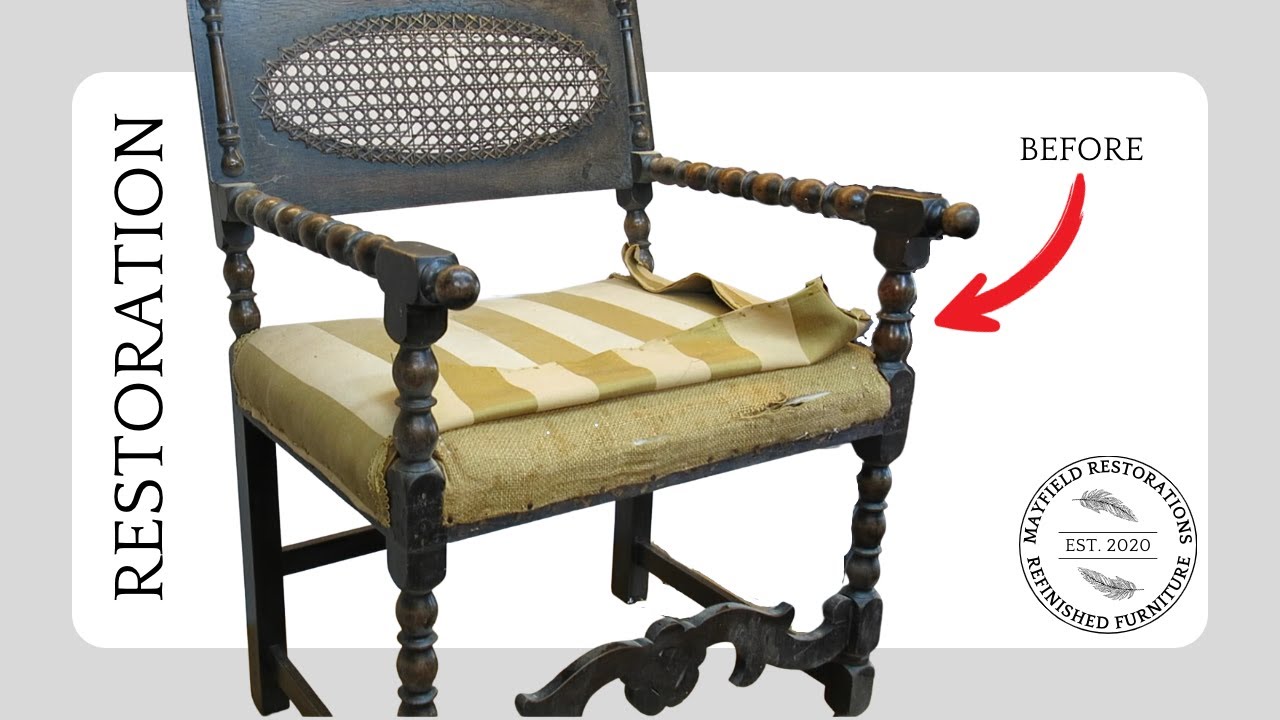The promotional photograph is a horizontally rectangular image with a gray border surrounding a white background. Centrally positioned to the left is an old wooden chair showcasing ornate carvings and a severely worn yellow and white striped cushion. The backrest of the chair features an oval mesh-like area, while the arms and front legs exhibit a twisty, bumpy texture; the back legs remain straight and dark brown. On the left side of the image, the word "Restoration" appears in a black and white background, and in the upper right corner, "Before" is written with a red arrow pointing towards the chair. At the bottom right, a circular logo reads "Mayfield Restorations, Refinished Furniture," flanked by two feathers, with "Established 2020" noted in the center.